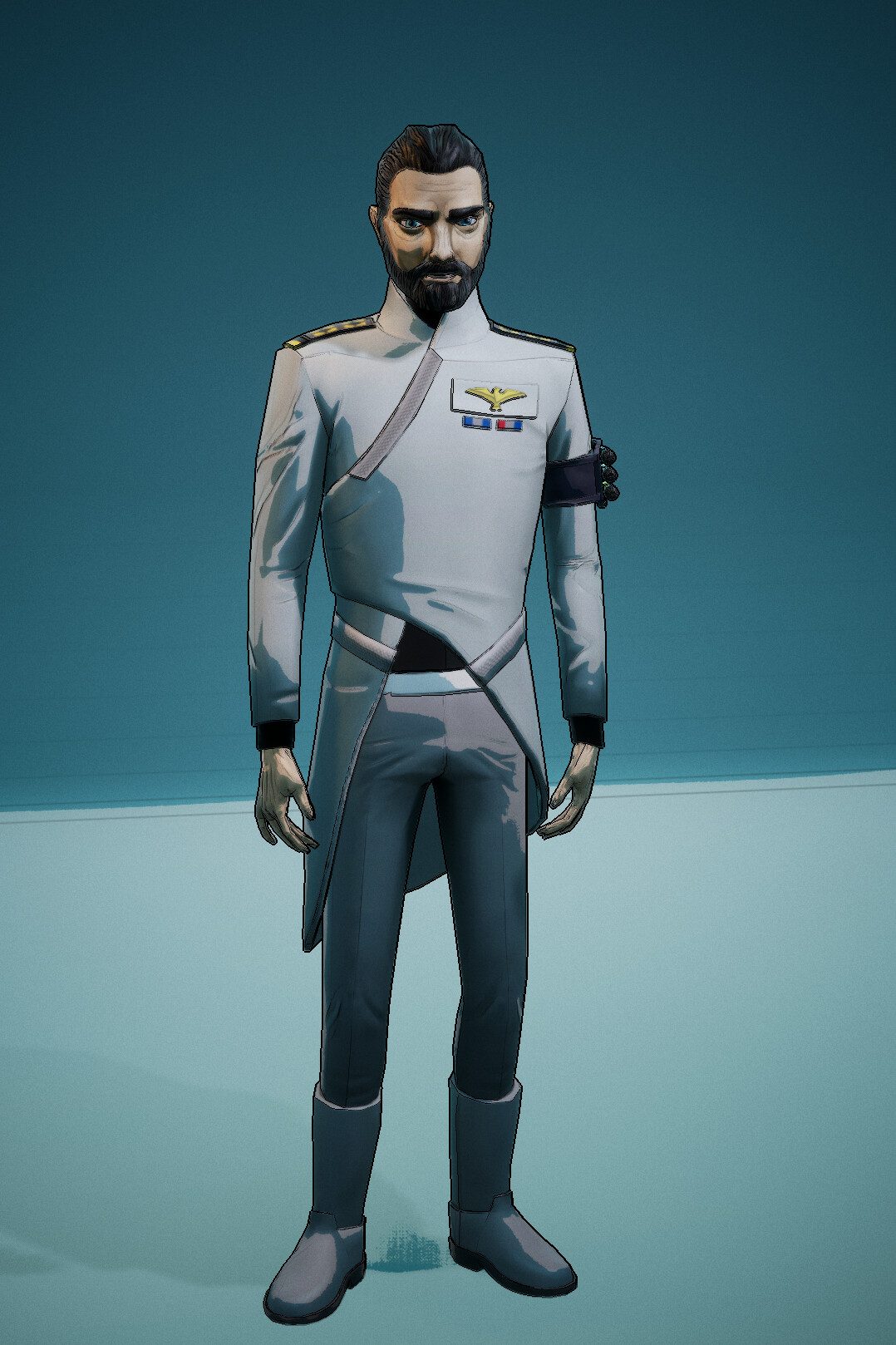The image displays a stylized depiction of a soldier against a multicolored blue background. The soldier, rendered in a cell-shaded artistic style, is seen wearing a long-sleeved gray jacket adorned with black cufflinks. Notable details include a golden eagle insignia prominently featured on the shoulders of his jacket, interspersed with stitched embellishments. He has gray hair and a gray beard, and his ensemble is completed with matching gray pants and boots. The overall impression is one of a stoic and distinguished figure, possibly representing a military persona from an unspecified country.